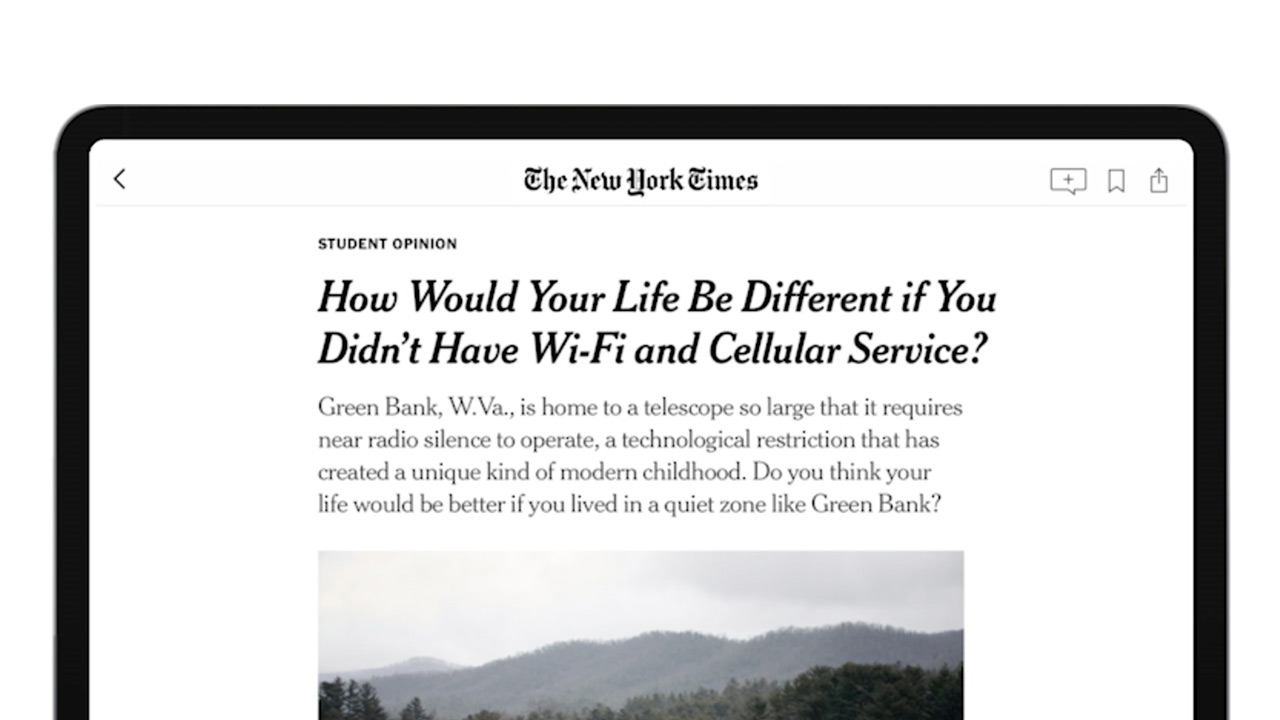This is a cleaned-up and detailed caption for the image:

---

The image is a screenshot of a New York Times article, prominently labeled under the "Student Opinion" section. The article's title, displayed in bold black text, reads: "How would your life be different if you didn't have Wi-Fi and cellular service?" Beneath the headline, the article begins by describing Green Bank, West Virginia (WVA), a town known for its enormous telescope that necessitates near radio silence, fostering an unusual modern childhood. The introductory text poses a thought-provoking question: "Do you think your life would be better if you lived in a quiet zone like Green Bank?"

In the top right corner of the screenshot, there are several interactive icons: a screen icon with a plus sign inside, resembling a speech bubble, a bookmark icon, and a share or download icon featuring an arrow exiting a box. Half-visible at the bottom of the screenshot is an accompanying image displaying a scenic view of a vast, verdant mountain range.

---